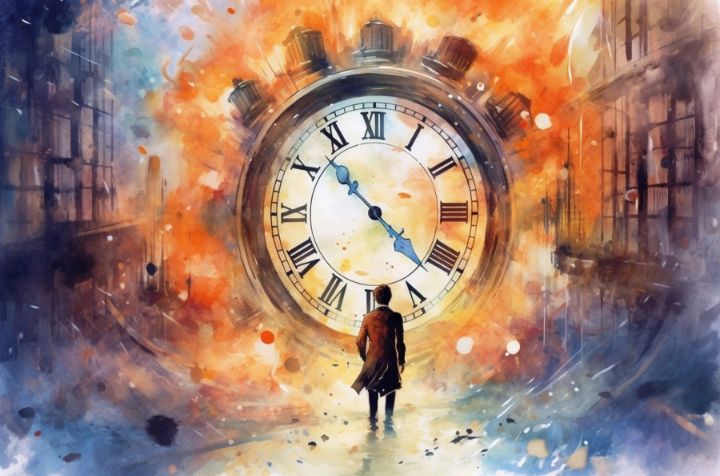The image appears to be a vivid, artistic creation, possibly inspired by a movie or a game. At the center stands a massive pocket watch with Roman numerals, its hands pointing to approximately 10:23. The clock face is a stark white with black numbering, and bluish-gray hands, topped by five metallic buttons. This grand timepiece is encircled by an explosive halo of flames rendered in a dynamic mix of reddish-orange, blue, and whitish hues, reminiscent of watercolor art. The scene is set within a loosely defined streetscape, with impressionistic buildings flanking either side. Positioned at the base of the clock, near the 6 o'clock mark, is a man with his back turned, intently gazing at the timepiece. He is dressed in a long brown overcoat, with a visible white collar and dark pants, his feet blending indistinctly into the ground below, suggesting either water or an unfinished aspect of the artwork. This evocative scene strongly echoes the dramatic flair of Dr. Strange or similar fantastical narratives.